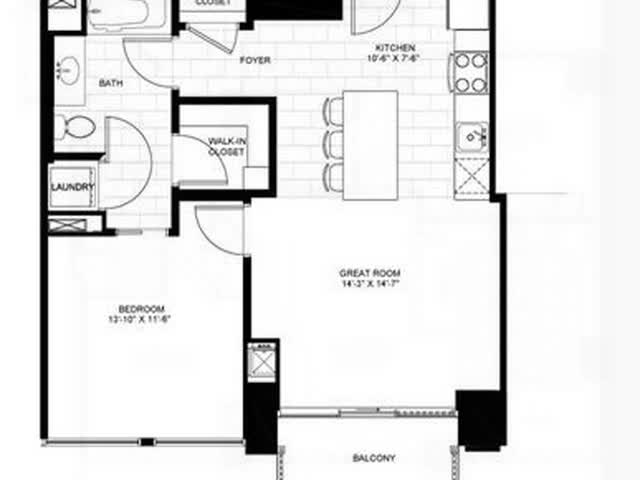The image depicts architectural plans for a house, outlined in black on a white background with varying line thicknesses to denote different elements. In the top left corner, a bathroom is situated, followed directly below by a laundry room and a walk-in closet. Adjacent to these rooms is a bedroom. Near the center-left of the plan is the entrance foyer, marked by a thick black line next to the doorway. 

To the right of the foyer lies the kitchen, complete with a stove top, sink, and a table with chairs. Below the kitchen, the space is labeled as the "great room," indicating it is the main living area. This room extends downwards to a balcony at the bottom of the plan. Flanking the great room and balcony on both right and left sides are thick black lines, potentially indicating storage spaces or structural elements.

Additionally, most of the rooms feature subtle horizontal and vertical lines, serving as a background grid or pattern, which is absent in the walk-in closet, bedroom, and great room.